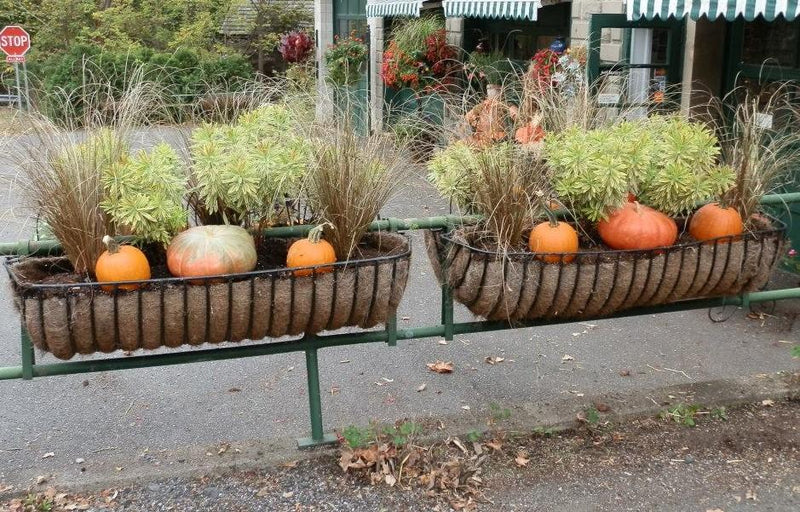The image captures a street scene featuring two large, oblong planters hanging against a green metal pipe fence. Each black metal planter, designed with visible strips, displays an arrangement of three pumpkins and some greenery, totaling six pumpkins in the image. In the upper left background, a stop sign is visible, surrounded by trees and foliage. To the right, a green and white awning marks the entrance to a retail space, likely a garden shop, as suggested by the open door. The ground is littered with leaves and some weeds, adding a touch of untidiness to the scene. There are no people present in the image.